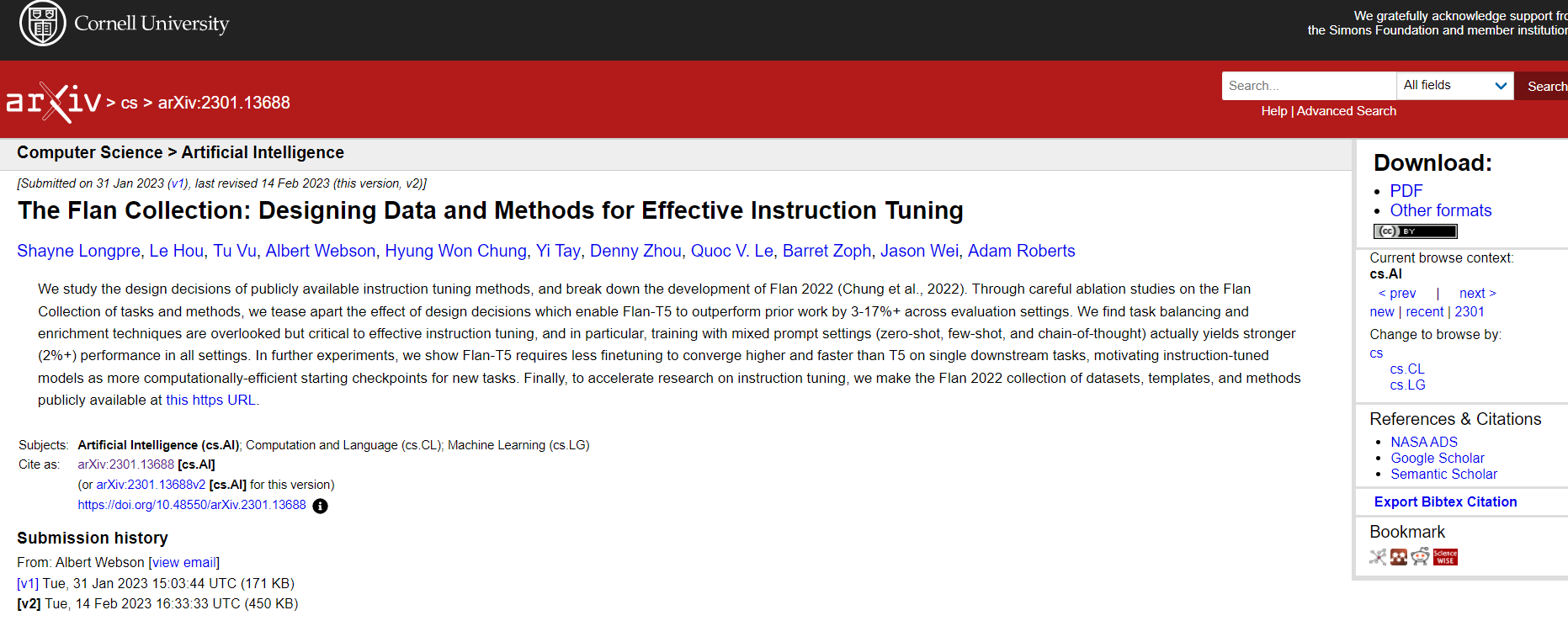A screenshot from the Cornell University website is displayed. At the top left corner of the page is the Cornell University logo, accompanied by the text "Cornell University." On the top right, there's a message stating "We gratefully acknowledge support in [unreadable details]." The entire top banner is black, followed by a red horizontal banner featuring various elements: "AR," a symbol resembling an 'X', "IV," an arrow pointing to "CS," another arrow, and some letters and numbers.

On the right-hand side of the red banner, there is a search box with a drop-down arrow beside it. Beneath this, the text "Computer Sciences" is displayed, with an arrow leading to "Artificial Intelligence." Below this section, an article begins, titled "The Flame Collection: Designing Data and Methods for Effective Instruction Tuning." Within the article, several names are highlighted in blue, indicating links. The main body of the article follows, ending with subject keywords, citations, and submission information.

To the right, a download section includes options for PDF and other formats, enabling the user to print the article in different formats.